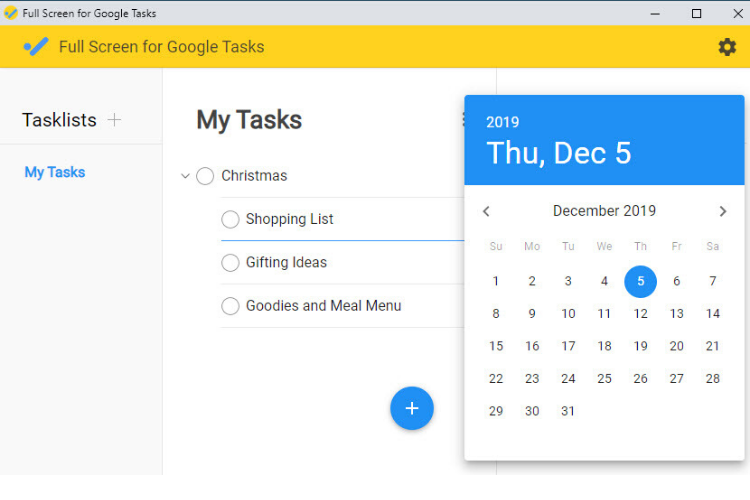This image showcases a detailed view of a web page interface designed for managing tasks and calendars. In the top left corner, a yellow circle contains a green checkmark, accompanied by text that reads "Full Screen for Google Task," extending from left to right. Adjacent to this is a black horizontal line, a black box, and a black 'X' icon.

The background below turns yellow, stretching across the screen, with a diagonal blue line intersected by a blue dot. Beside the blue dot, there's another label that reads "Full Screen for Google Cast Task." To the right of this label, there is a settings icon depicted as a gear.

As we move lower on the page, there's a gray background area on the left labeled "Task List." Beneath this heading, the text "My Task" appears in blue, and to the right on a white background, it is repeated as "My Task." Below this white section is a vertical list comprising four circles aligned from top to bottom. The labels adjacent to these circles are (from top to bottom): "Christmas," "Shopping List," "Gifting Ideas," "Goodies and Meal Menu." Below this list, there is a blue circle featuring a white plus sign.

To the right side of the "My Task" section, there is a calendar. The calendar's header is blue, displaying "2019" and "Thursday, December 5th." The main body of the calendar is white, showing the days of the month. Navigation arrows appear on the left and right, allowing users to move between months. The specific date, December 5th, is circled in blue.